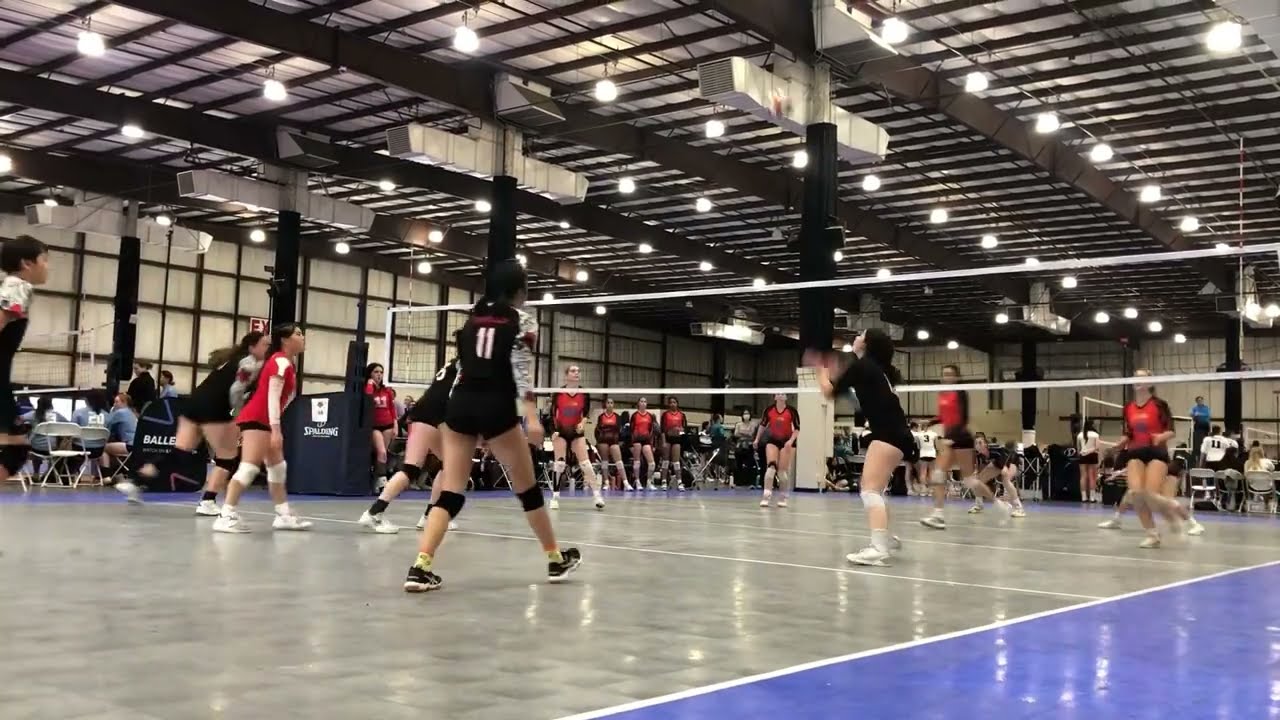In a vast, brightly lit gymnasium resembling an aircraft hangar, a thrilling women's volleyball match unfolds on a smooth, reflective floor. The arena is alive with action as players from the black-uniformed team, positioned nearest to the camera, engage in mid-motion against their red-uniformed opponents across the net. One player in red seems to be temporarily on the black team's side, suggesting a casual or adaptive team arrangement. The focus is on a player in the center, knees bent, hands outstretched, prepared to make a play, while her teammates gaze upward, indicating the ball's imminent descent. Surrounding the court, spectators and additional teams in light blue are seated and standing, adding to the lively atmosphere of this indoor sports complex. Bright overhead lights illuminate the scene, casting reflections on the polished, marble-like floor as the game progresses with dynamic intensity.